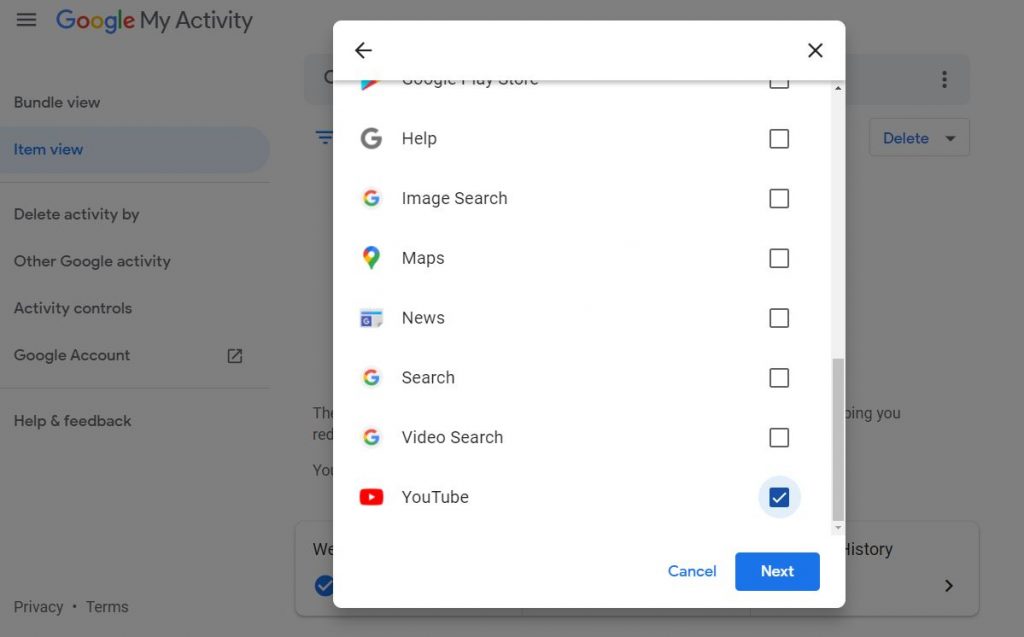The image is a detailed screenshot of a Google Activity page displayed in the background. In the top left corner, there are three horizontal lines followed by the label "Google My Activity." Below this heading, on the left-hand side, there are several options listed in a grayed-out format: "Bundle View," "Item View," "Delete Activity by," "Other Google Activity," "Activity Controls," "Google Account," "Help and Feedback." The "Item View" option is currently highlighted.

Superimposed over this background is a bright white overlay screen featuring a list of options with checkboxes next to them. The first option's label is obscured, while the subsequent options are "Help," "Image Search," "Maps," "News," "Search," "Video Search," and "YouTube." The checkbox next to "YouTube" is ticked. At the bottom of this overlay, there are two blue buttons: "Cancel" and "Next."

On the right side of the image, the background screen shows a visible dropdown menu labeled "Delete." Additionally, at the bottom of the entire composite image, there's a square with a checkmark on the left and a forward arrow on the right; the partial word "History" is visible within this box. In the bottom left-hand corner of the background screen, the labels "Privacy" and "Terms" can be seen. At the top of the superimposed overlay, there are icons for a back arrow and an 'X' to close the overlay.